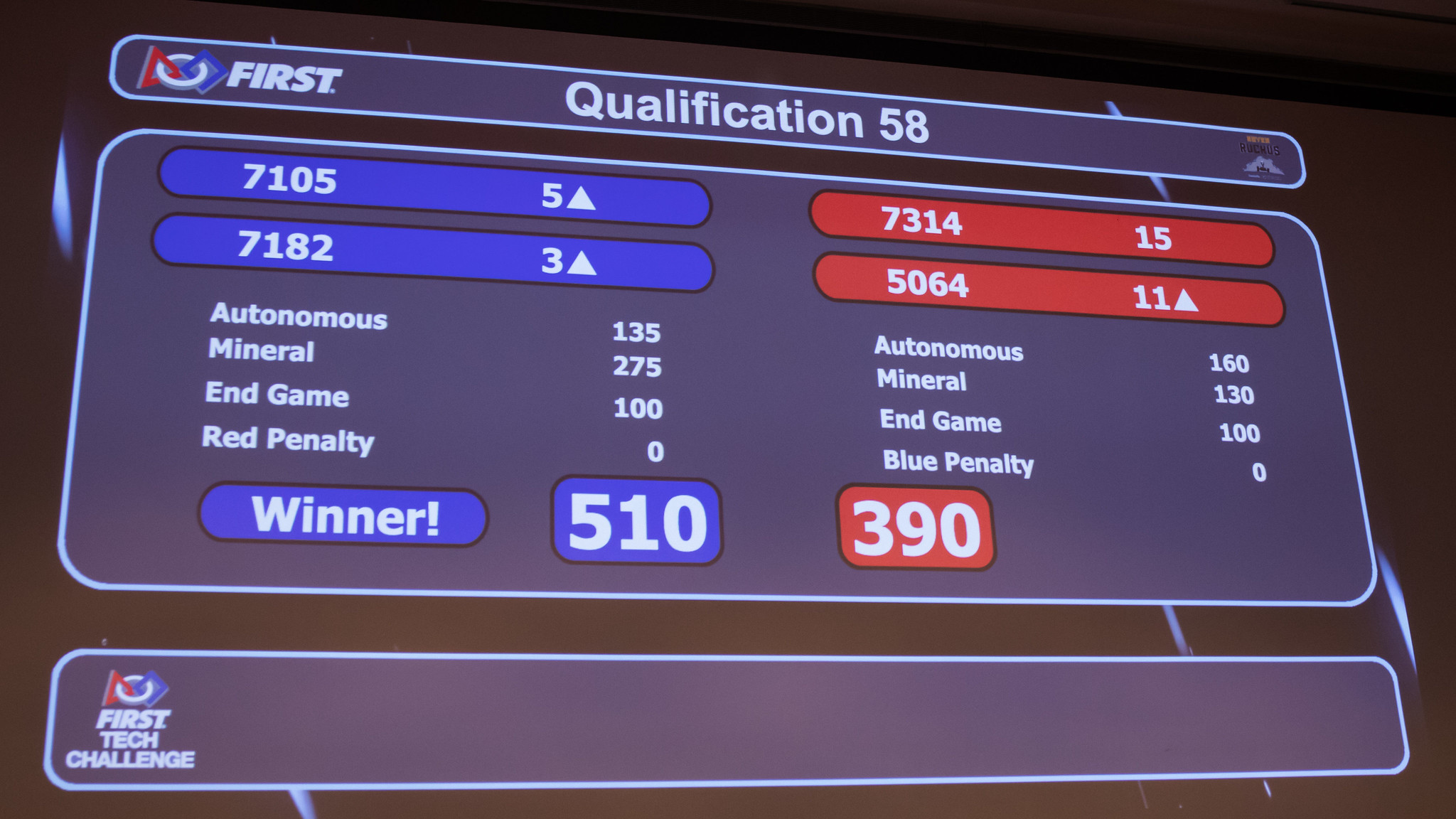The image depicts a black-background scoreboard used in a sports broadcast, specifically for the "FIRST Tech Challenge," which is noticeable from the logo at the top—featuring a red triangle, a white circle, and a blue diamond intersecting. At the top, it reads "FIRST Qualification 58" in white text within a dark blue rectangular section bordered by light blue. 

The scoreboard is divided into two identical columns, representing two competing teams. The left column is for the blue team with identifiers 7105 (5) and 7182 (3), and the right column is for the red team with identifiers 7314 (15) and 5064 (11). Key statistics for each team are listed below their identifiers:

- For the blue team:
  - Autonomous: 135
  - Mineral: 275
  - End Game: 100
  - Penalty: 0

- For the red team:
  - Autonomous: 160
  - Mineral: 130
  - End Game: 100
  - Penalty: 0

At the bottom of the scoreboard, a blue box with white text declares the winner, listing the blue team with a final score of 510, compared to the red team's score of 390.